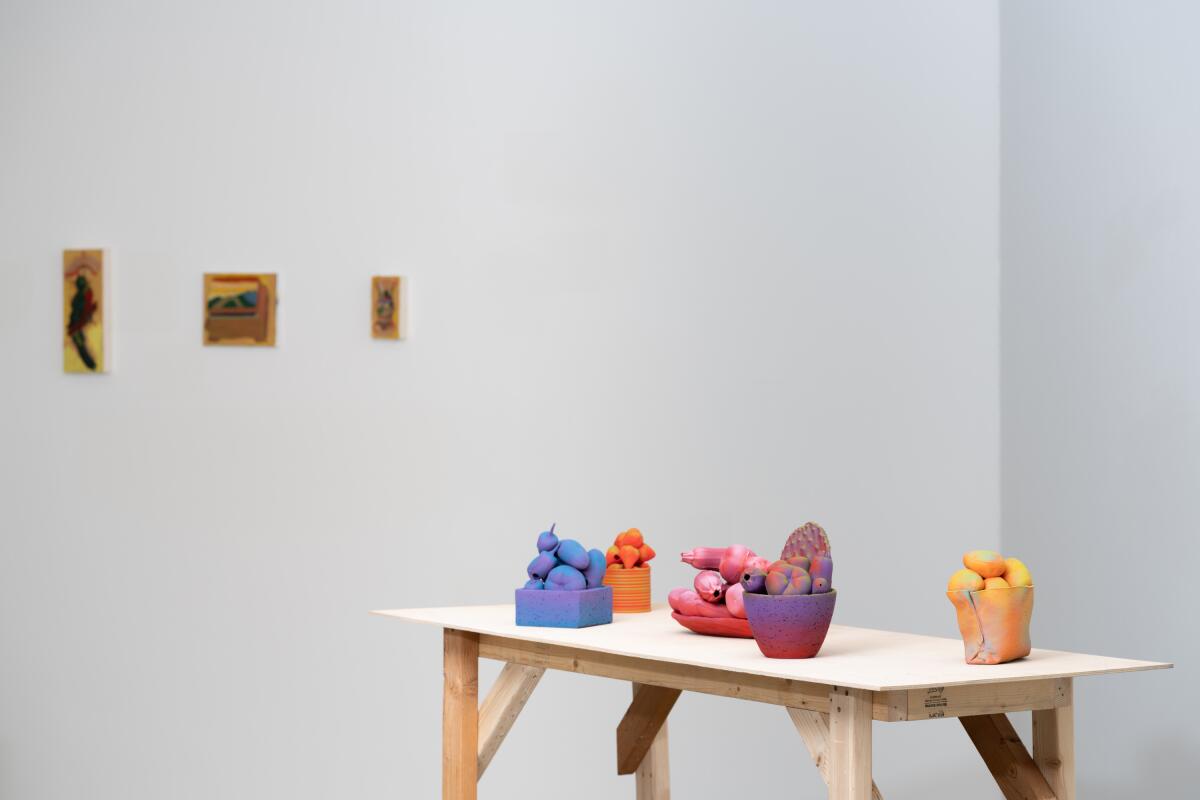The image depicts a sparsely furnished room with white walls. The primary focus is a roughly constructed table positioned at the bottom right corner of the image. The table, appearing homemade, is made from a thin sheet of plywood supported by several 2x4 planks, with additional diagonal planks reinforcing the legs. On top of the table are five distinct artistic bowls and containers, each seemingly filled with fruit-like objects in various colors. To the right, there's an orangish-yellow bowl containing mangoes. Towards the middle-left of the table is a reddish bowl that transitions to purple, holding a mix of fruit-like items. There is also a shorter, longer red bowl with red fruit. Additionally, a bluish-purple box holds blue oval fruits, while further to the left, an orange jar or box holds orange fruits. Hanging on the left wall, about halfway up, are three small, predominantly yellow paintings featuring brown and black drawings. The room is bare, accentuating the simple yet colorful arrangement on the table.